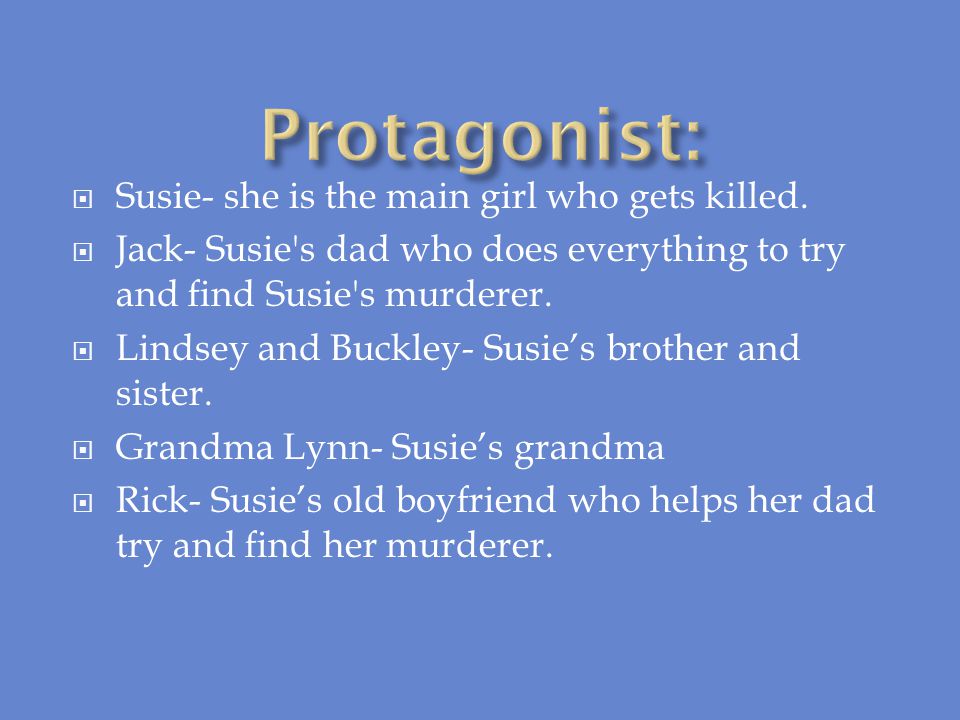The image is a potential slide for a PowerPoint presentation featuring a solid blue background. The top middle of the image displays the title "Protagonist:" in large, yellow text with a drop shadow effect. Below the title, there are five bullet points, each represented by a tiny square within a larger square, all in white text. The first point describes Susie, the main girl who gets killed. The second point introduces Jack, Susie's dad, who does everything to try and find Susie's murderer. The third point includes Lindsay and Buckley, Susie's brother and sister. The fourth point is about Grandma Lynn, Susie's grandma. The final point mentions Rick, Susie's old boyfriend, who helps her dad try and find her murderer. There are no additional images on the slide.